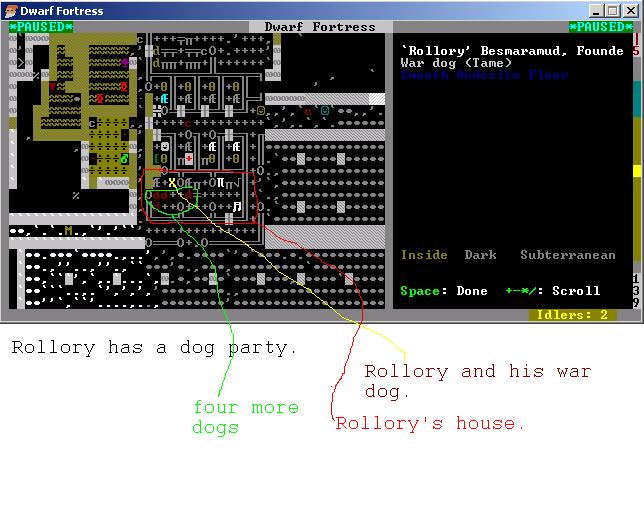The image is a detailed screenshot in landscape orientation of a game window from the old-school game "Dwarf Fortress", reminiscent of a Windows 3.1 or Windows 95 interface. The upper section features a prominent blue banner running across the top with "Dwarf Fortress" written in white text on the left side and a set of traditional navigational buttons (minimize, expand, and close) on the right. Just below this banner in the upper left corner, the game status is displayed as "paused" in green, accompanied by a small dwarf icon.

The main section of the image is divided into two parts. The left two-thirds showcase a top-down, 8-bit style maze that conjures images of the game "Legend of Zelda" or the board game "Clue". This maze is composed of black and gold pathways leading through various rooms. Specific areas and characters are marked with colored lines and text, such as "Rollery and his Wardog" in yellow and "Rollery's house" outlined in red. At the bottom of this section, a gray bar stretches from left to right with the text "Idlers: 2".

The right one-third of the image is occupied by a black chat box displaying white text commentary about the game's action. At the top of this section, additional text strings such as "file minus" and character dialogues are visible, followed by a detailed status report, including a character named "Rollory Besmaramud" and a "Wardog (tame)". The chat box closes with game environment details like "inside dark subterranean" and navigational commands such as "done + - * / ; scroll". Below this, the narrative includes lines pointing out "Rollery has a dog party" with "four more dogs" highlighted in green.

Overall, the scene is a nostalgic, pixelated depiction of a paused game screen, illustrating both the in-game map and running commentary in classic retro gaming style.